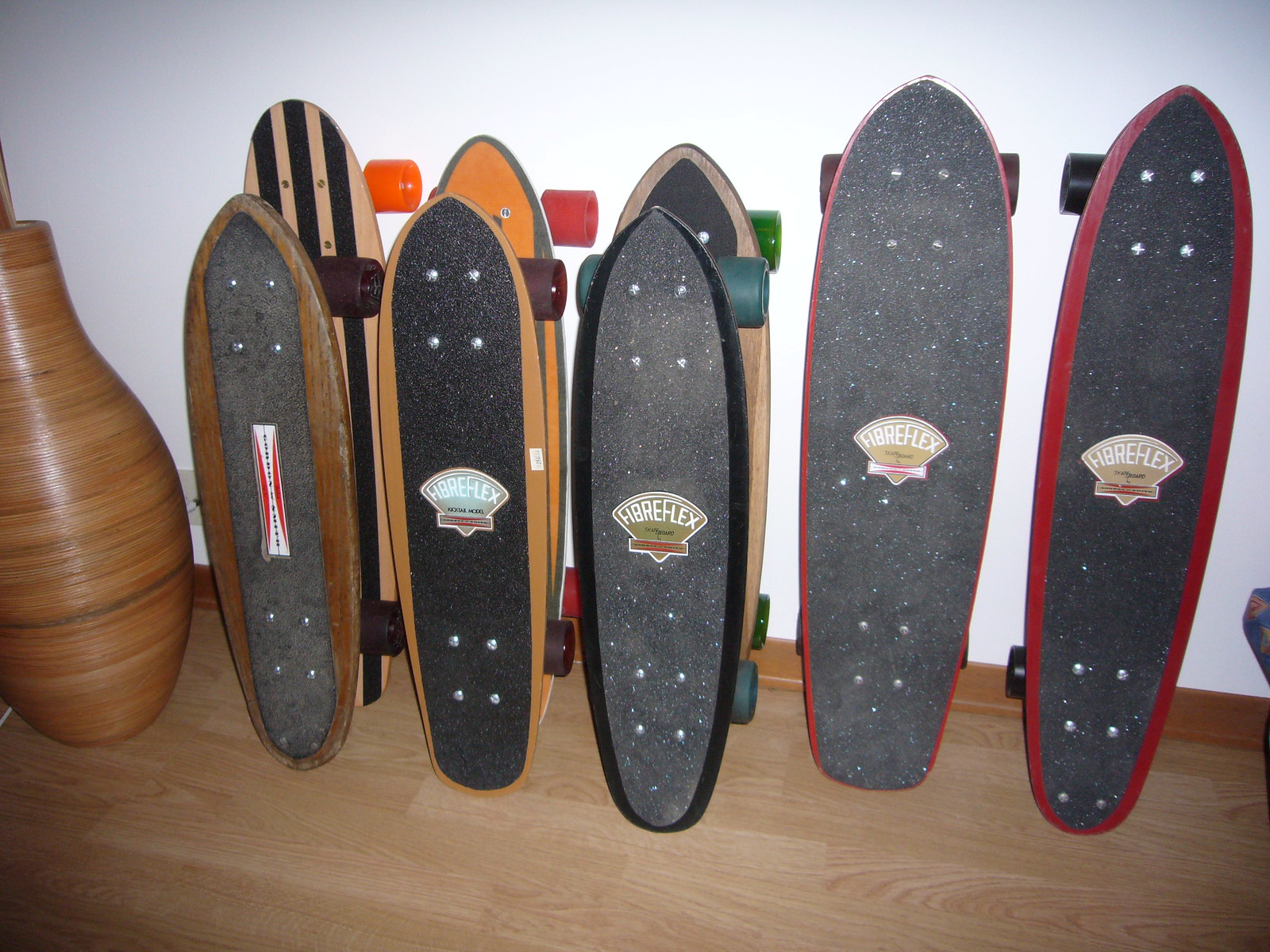The image depicts a well-lit indoor scene with eight skateboards arranged on a light brown wooden floor against a white wall. To the far left, there is a tall, brown pottery vase about the same height as the skateboards, possibly resembling Native American craftsmanship. Among the skateboards, six are grouped closely together on the left, while two larger ones are slightly apart on the right.

On the left, a black and white vertically striped skateboard with orange wheels stands at the back, followed by a brown wood skateboard with a black sandpaper-like center. An orange skateboard with gray trim and red wheels is next, paired with another brown-trimmed skateboard featuring a black sandpaper-like material in the center and a label with "FiberFlex." Beside these, a beige and black board with green wheels sits, along with another black-trimmed one also labeled "FiberFlex."

On the right, the larger skateboards are each trimmed in red, featuring black wheels and the recognizable black sandpaper-like center, also branded with "FiberFlex." The skateboards exhibit a variety of wheel colors, including orange, red, purple, teal, green, black, and dark brown, adding a colorful contrast to the uniform wooden floor and white wall.